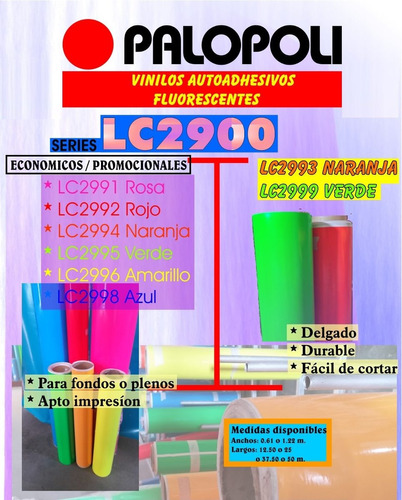The image features a vibrant advertisement, primarily in Spanish, displaying a product named "PALLOPOLI," prominently written in black uppercase letters at the top center, accompanied by a distinctive red circle to its left. Below the title, a red horizontal rectangle contains yellow text that reads "Vinilos Autoadhesivos Fluorescentes." Right under this, a shorter blue rectangle houses the lettering "LC2900" in a light silvery-pink hue. The lower left corner of this blue rectangle features a thin smaller blue rectangle with the word "SERIES" in black. 

Center-left, a series of vertically aligned text displays various colors corresponding to actual text colors: LC2991 in purple (Rosa), LC2992 in red (Rojo), LC2994 in orange (Naranja), LC2995 in green (Verde), and LC2996 in yellow (Amarillo). Below these, black text reads "para fondos o plenos" and "apto impresión."

On the right side, starting mid-image, "LC2993 Naranja" and "LC2999 Verde" are listed in yellow and green within a yellow rectangle with a dark orange border. Below them are images of green and red rolls. 

Additionally, three small yellow rectangles under the rolls have black starred texts: "DELGADO," "DURABLE," and "FACIL DE CORTAR." More pale colored rolls—yellow, blue, and green—are horizontally aligned below. The image includes another yellowish roll at the bottom right corner with measurements in a blue and orange bordered rectangle stating "MEDIDAS DISPONIBLES" and specific dimensions.

In the bottom left corner, more brightly colored rolls, including blue, red, and purple, stand vertically, with shorter green, orange, and yellow rolls in front. The overall backdrop is a light purplish-gray color resembling a desktop setting, emphasizing the array of colorful self-adhesive fluorescent vinyl rolls available for various uses.